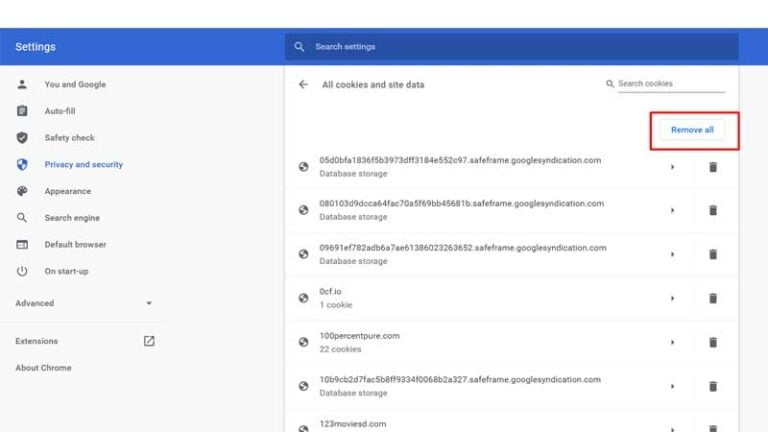The image showcases a settings window divided into two primary sections: a vertical menu on the left and the main content area on the right. A blue bar spans the top of the window, indicating "Settings" on the left side and featuring a search bar labeled "Search settings" on the right side. 

In the left-hand vertical menu, the "Privacy and settings" option is selected. The right-hand main content area focuses on cookie management, displaying the heading "All cookies and site data" at the upper left. Below this heading, a prominent "Remove all" button, outlined in red, allows users to delete all cookies listed. The current list shows seven cookies that can be removed using this option.